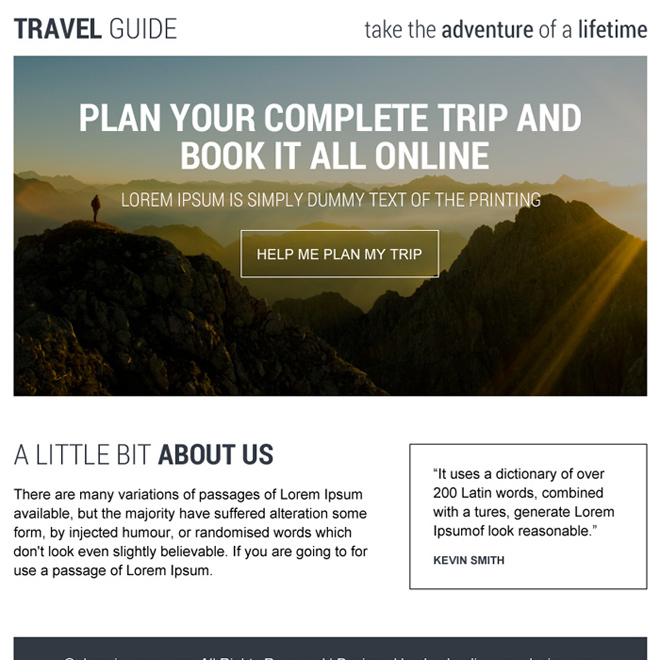Screenshot of a travel guide webpage. At the top, there's a white navigation bar featuring "Travel Guide" on the left and "Take the Adventure of a Lifetime" on the right. Backgrounded by a stunning image of tall mountains, a lone adventurer stands on a peak to the left. Superimposed over this landscape, large white text reads, "Plan your complete trip and book it all online." Below, smaller text says, "Lorem Ipsum is simply dummy text of the printing." A prominent button labeled "Help Me Plan My Trip" sits beneath this text. The lower section of the screenshot is divided into two columns. The left column, titled "A Little Bit About Us," contains placeholder text: "There are many variations of passages of Lorem Ipsum available, but the majority have suffered alterations in some form."